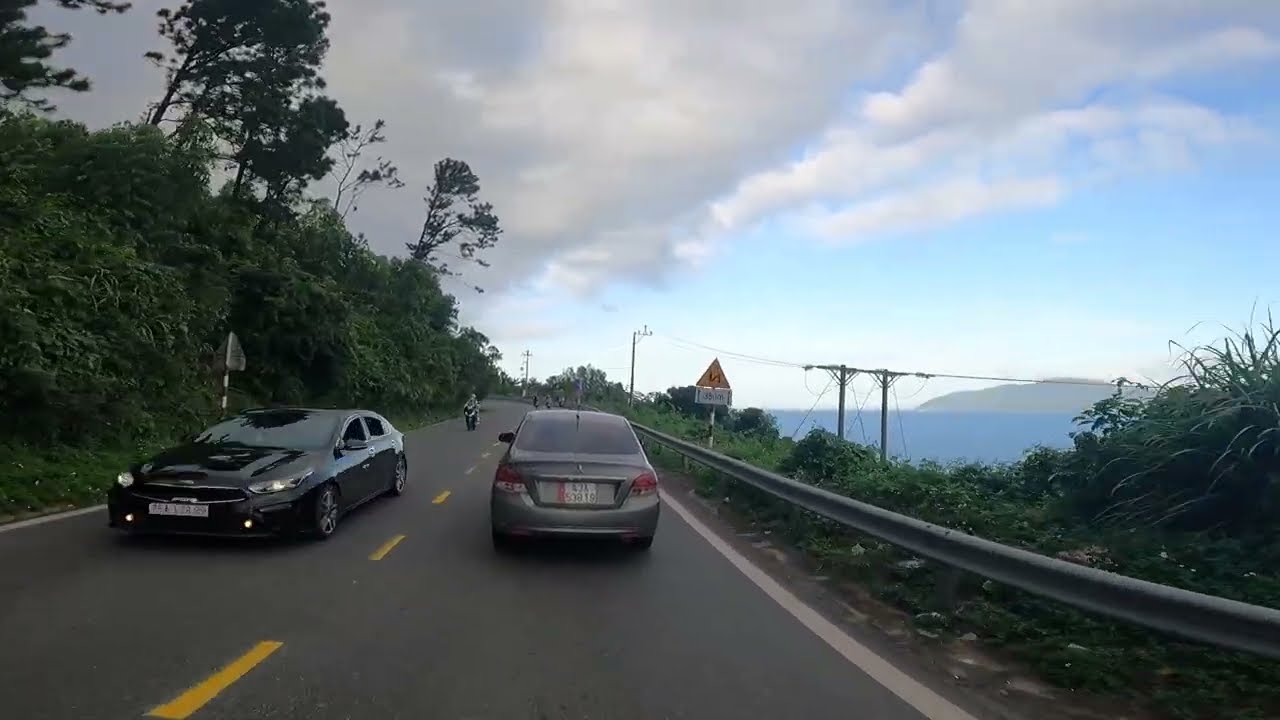This photograph, approximately six inches wide and three to four inches tall, captures a daytime scene on a straight road that curves slightly to the left further ahead. The image is taken from the right-hand lane of a two-lane road. Directly in front is a gray sedan, and to the left, a four-door black sedan approaches in the opposite direction. A bike is also visible on the road.

The road delineations include a solid white line to the right, beside a gray metallic barrier, and a yellow dotted line separating the two lanes. The right side of the road is bordered by a metallic fence beyond which lies green foliage, brush, and a cliff edge. On this side, there are signboards and a power line extending into the distance. One sign features a yellow triangle with a black zigzag mark.

Beyond the barrier and foliage on the right, the terrain drops off to reveal a large blue water body, possibly an ocean or bay inlet, with a hill or mountain in the background. The left side of the road transitions into green plants, trees, and a grassy hill, presenting a landscape of natural greenery.

The sky above is a mix of blue with some darkening clouds, especially towards the upper left corner, adding a dynamic weather element to the serene outdoor setting. The combination of natural and manmade elements converges in this detailed snapshot of a bustling roadside scene.